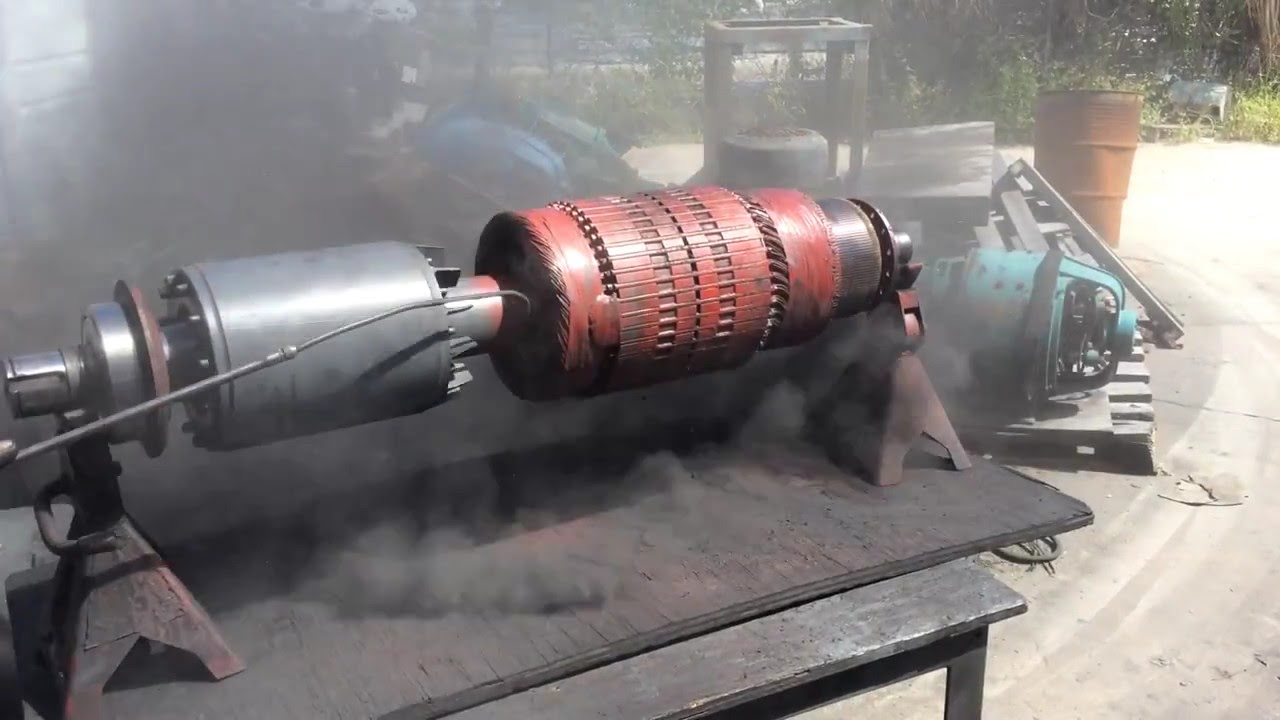The image features a large, intricate piece of mechanical equipment, likely part of an engine, situated outdoors on a gray surface. The machinery is notably cylindrical, with a rounded, dark red central section and a gray section featuring several spikes. It's supported by two red and brown metal legs and seems to rest on a black slab on top of a table. The surrounding scene includes various mechanical objects, facilitating an industrial ambiance with additional engine parts and rotors scattered around. There's evident rust on the barrel in the background amidst a grassy, tree-filled area, all under daytime light. Smoke emanates from the equipment, indicating it might be operational. Additionally, there's an aqua blue piece of machinery visible to the left. The ground surrounding the area is light tan, contributing to the rugged, outdoor setting.